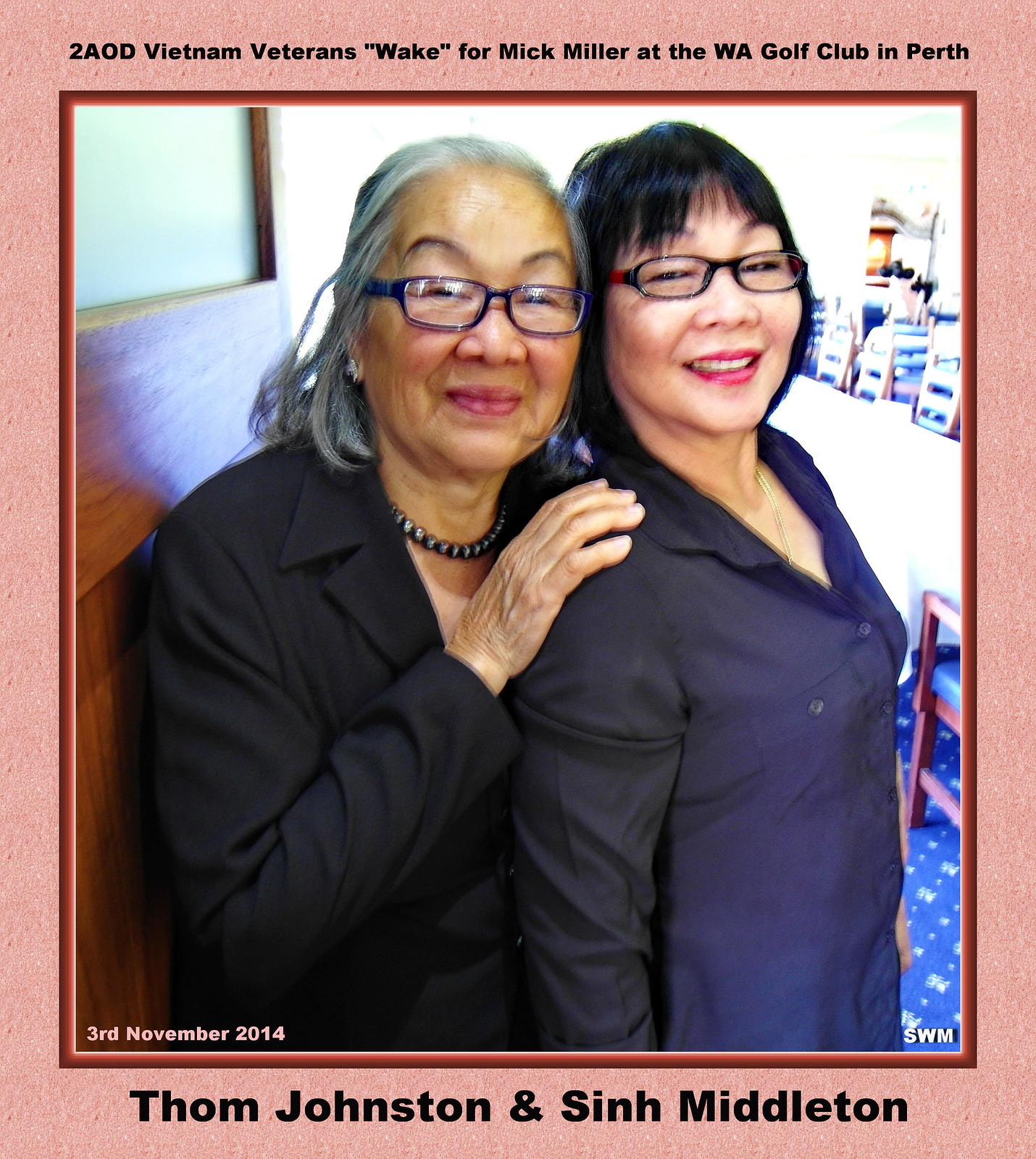The photograph, taken on November 3, 2014, depicts two Asian women, possibly related as mother and daughter, against a wood-colored door at the WA Golf Club in Perth during a wake for Vietnam veteran Mick Miller. The woman on the left appears to be in her 60s or 70s, dressed in a navy button-up shirt and glasses, while the woman on the right, seemingly in her 50s or 60s, wears a black button-up shirt, glasses, and a black necklace. The older woman places her hand on the younger woman's shoulder, suggesting affection or support. Both names on the image, Tom Johnston and Sin Middleton, could represent them. The photograph features a post-production red and pink speckled border with an additional brown and orange frame. In the blurred background, there are hints of blue and white colors and a brown-framed chair.